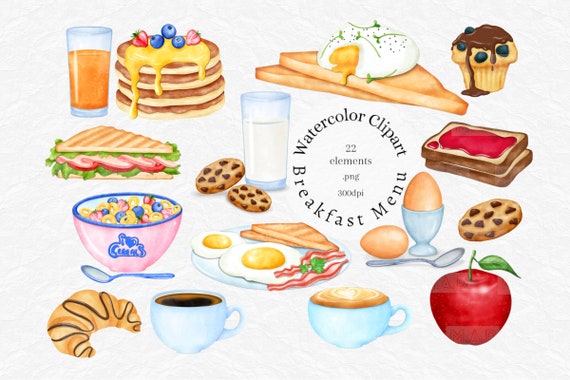This image is a detailed watercolor clipart of a breakfast menu with 22 elements, rendered at 300 DPI. Central to the composition is the text "Watercolor Clipart 22Elements.png 300 DPI Breakfast Menu," encircled by various types of breakfast food items. The assortment includes a glass of orange juice, a stack of pancakes topped with syrup, butter, and berries, a poached egg with a runny yolk, and a blueberry muffin covered in chocolate sauce. There's also a sandwich likely filled with lettuce and tomatoes, two chocolate chip cookies paired with a glass of milk, and toast smeared with raspberry jam. Additional items include a bowl of colorful cereal rings labeled "I love cereal" with a spoon at its side, a croissant with chocolate icing, a cup of plain coffee, as well as a cup of coffee with latte art. A breakfast plate features fried eggs, bacon, parsley, and white toast, accompanied by a glass of milk. There's another set of two cookies, toast, boiled eggs in and out of egg cups with a silver spoon, and finally, a vivid red apple. This comprehensive and artistically styled collection of breakfast items could serve as a charming decorative set for digital or printed use.